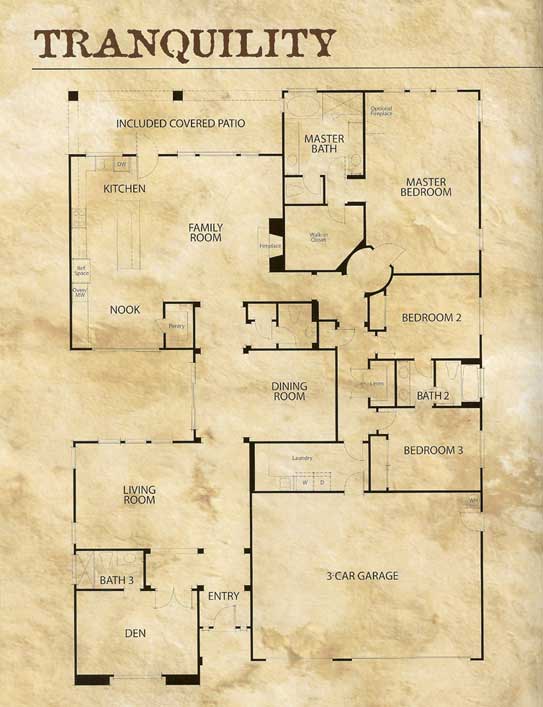The image showcases a vertically-oriented floor plan set against an antique, tie-dyed background featuring a blend of yellowy-tan, creamy-beige hues. The backdrop mimics an old-fashioned texture with visible crinkles and waviness, lending a sense of depth and character. 

At the top of the floor plan, the word "TRANQUILITY" is boldly displayed in uppercase brown letters, intersected by a horizontal line stretching towards the right. The detailed floor plan below comprises various rectangles and squares, carefully delineating the layout of a home. 

Key elements of the floor plan include:

- **Covered Patio**: Positioned at the top, clearly labeled in uppercase black letters.
- **Kitchen and Family Room**: Located centrally, with adjoining areas marked as "nook" and "pantry" below the kitchen.
- **Master Suite**: Situated in the upper right corner, featuring a master bathroom, bedroom, and closet.
- **Bedrooms and Bathrooms**: Bedroom two leads into a second bathroom, which in turn leads to bedroom three, indicating a shared Jack and Jill layout.
- **Laundry Room**: Positioned to the left of bedroom three.
- **Three-Car Garage**: Located at the bottom of the page, indicating ample parking space.

The intricate floor plan offers a comprehensive depiction of the home's layout, combining practical design with an aesthetically pleasing, textured background.